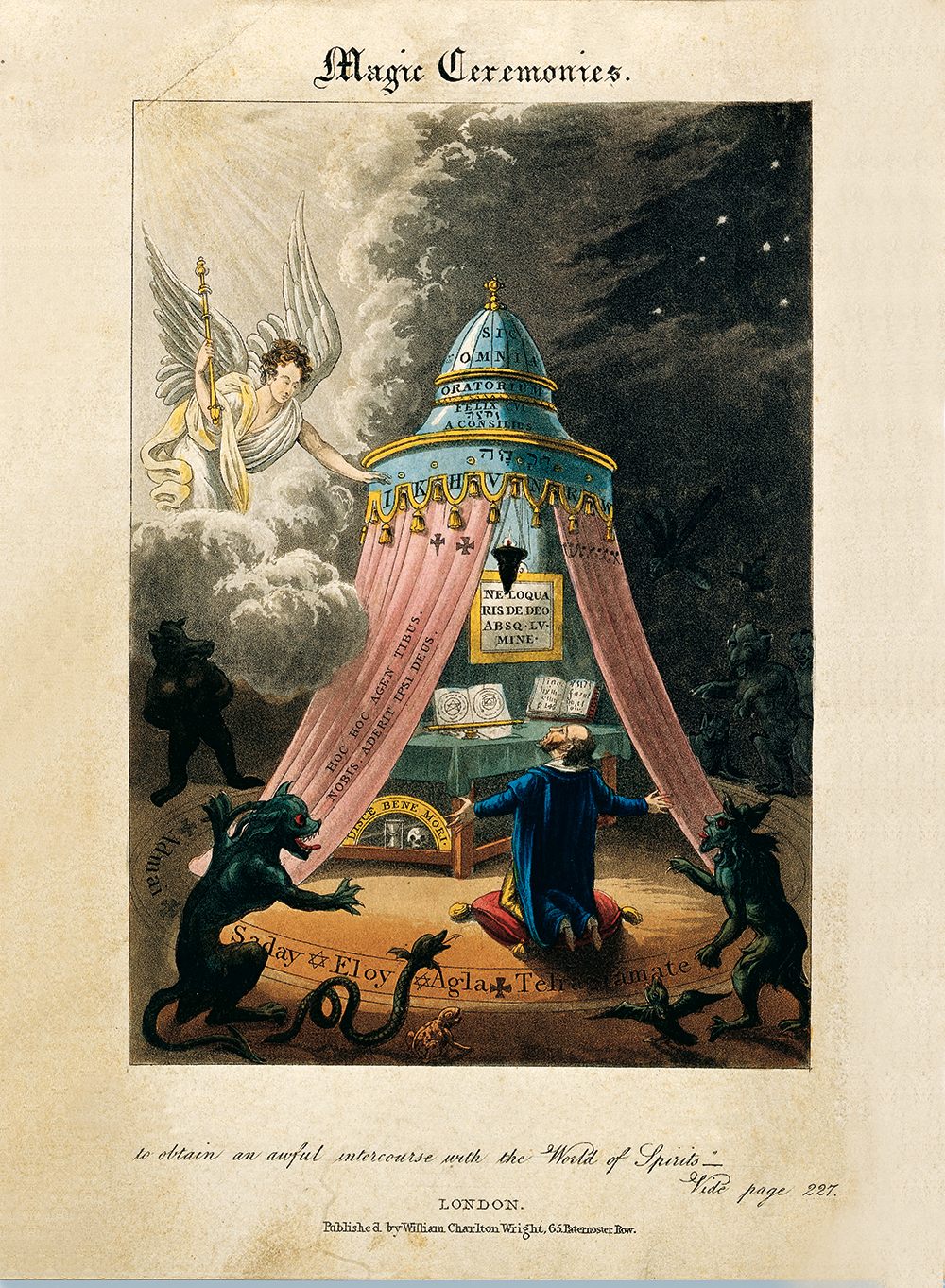This image appears to be an old, intricately designed poster or page, possibly from a historical book. The outer edge of the page is a faded tan or yellowish paper with dark brown spots, adding to its aged look. At the top, in a fancy font, are the words "Magic Ceremonies." The bottom of the poster reads, "To obtain an awful intercourse with the world of spirits, page 227, London," though part of the publishing information is blurred.

The scene depicted in the image is set under a dark night sky dotted with stars. Central to the image is a tent-like structure with a dome, adorned with a blue and yellow top and red curtains. Inside the dome, Latin-like writing is visible on a poster. A red cushion sits on the ground, supporting a man clad in yellow pants and a blue jacket, kneeling with outstretched arms, seemingly in prayer or supplication. A greenish tablecloth covers a table that holds several books.

In the foreground, menacing demons with bulging red eyes, lapping tongues, and long curly tails surround the man. There appear to be three such demons, along with eerie snakes and ominous birds circling him. On the left side of the image, a luminous angel holding a staff descends from a puffy cloud, casting a divine light on the man below, creating a stark contrast with the encroaching darkness and demonic figures on the right side. The detailed and vivid depiction suggests a scene of spiritual conflict, as the man seems to be praying for salvation from the surrounding dark entities.